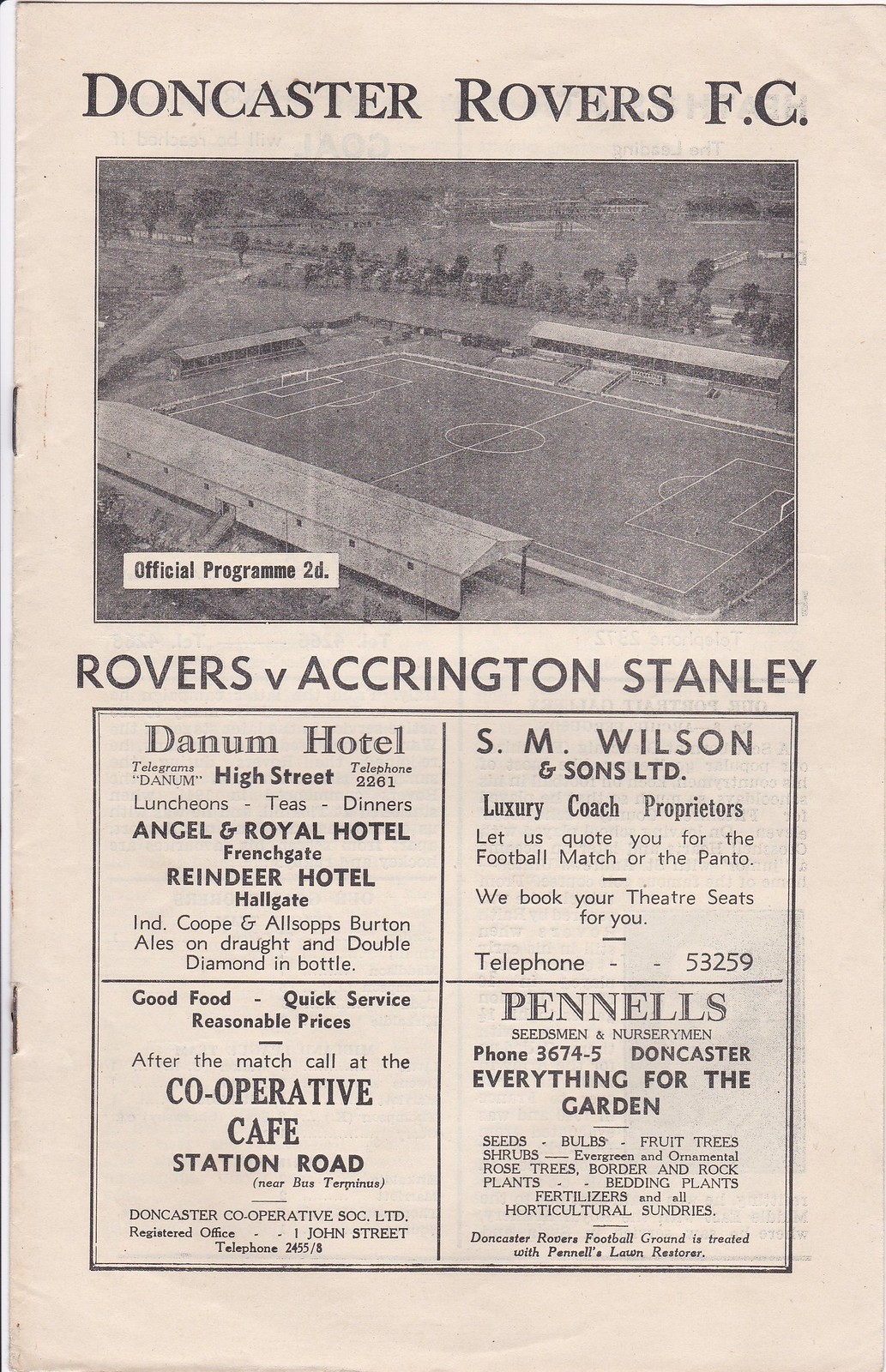The image is a vintage, black-and-white soccer program that appears to be very old, with a cream-colored aged background. At the top, in bold black letters, it reads "Doncaster Rovers FC." Below that is a high-angle, black-and-white photograph of a soccer field, labeled "Official Program 2D," indicating it is an official game program. The matchup is noted as "Rovers vs. Accrington Stanley." The bottom section of the program features advertisements and sponsor information, divided into four distinct boxes. In the top left box, there is an ad for Danum Hotel, promoting lunches, teas, and dinners along with beverages. The top right box displays an ad for S.M. Wilson & Sons Ltd., offering luxury coach services and theater seat bookings. The bottom left box advertises the Cooperative Cafe on Station Road, highlighting good food, quick service, and reasonable prices, and encourages visitors to drop by after the match. The bottom right box features Pennell's Seedsmen and Nurserymen, promoting gardening supplies and services with the contact phone number 36745 Doncaster.